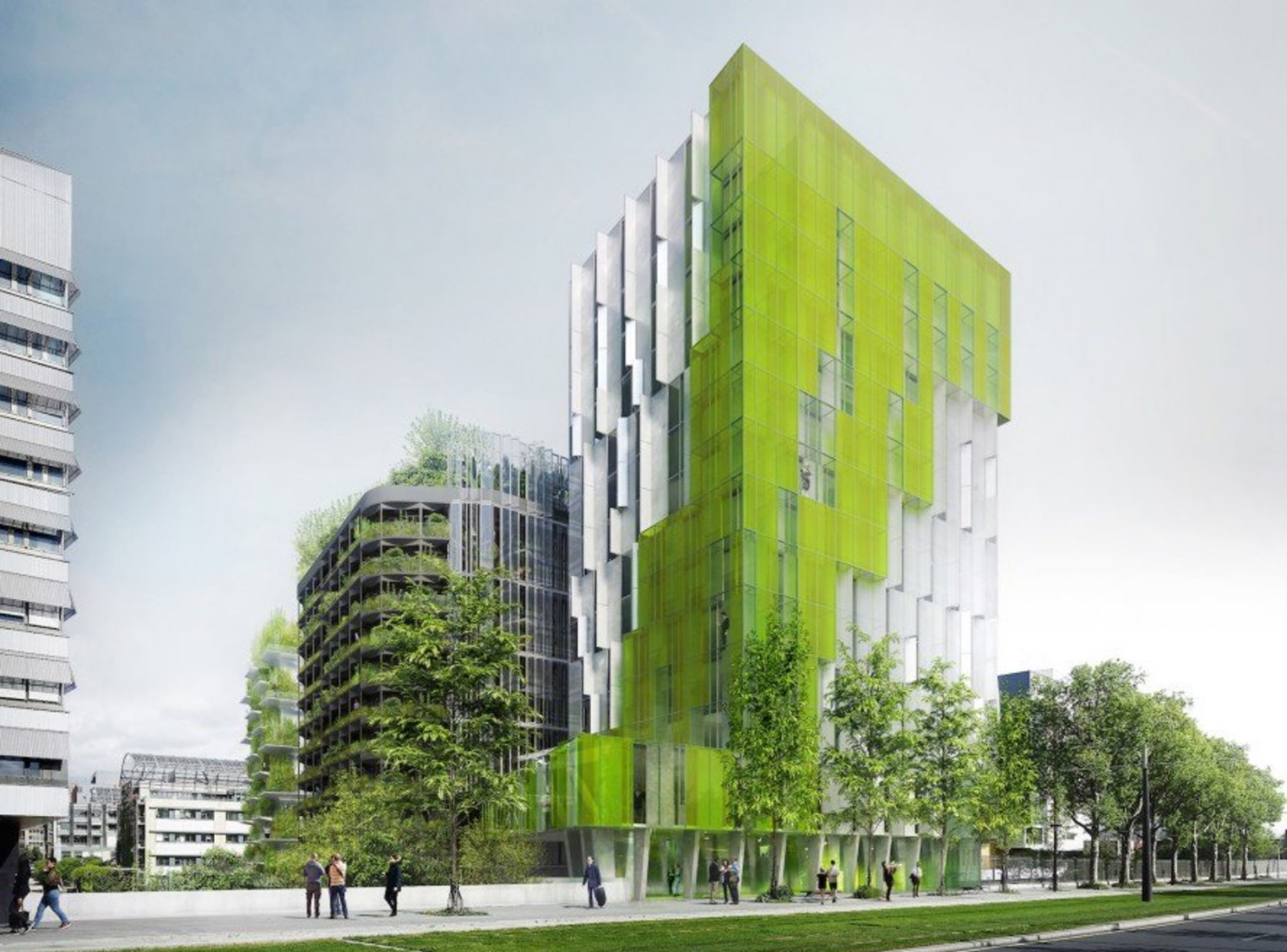The image depicts a computer-generated or artist-rendered scene of a futuristic urban landscape. The central focal point is a large, geometrically-shaped, white rectangular building adorned with translucent lime-green glass panes that allow light to filter through. This building is surrounded by numerous rectangular windows and is bustling with activity; various individuals populate the scene, including one person taking a picture, pairs of people walking and talking, and some entering or leaving the building. 

Adjacent to this central structure is another tall gray building, reminiscent of a parking garage. This second building is enveloped in abundant greenery, with plants cascading over multiple levels and even sprouting from the rooftop, creating an almost post-apocalyptic, overgrown atmosphere. 

In the foreground, the street is framed by a grassy area and a sidewalk lined with trees, where more people are gathered. Additional buildings can be seen in the background, including another large white and gray structure that lacks the same level of vegetation. The sky above is a mix of light blue and white, enhancing the serene yet vibrant energy of the scene.